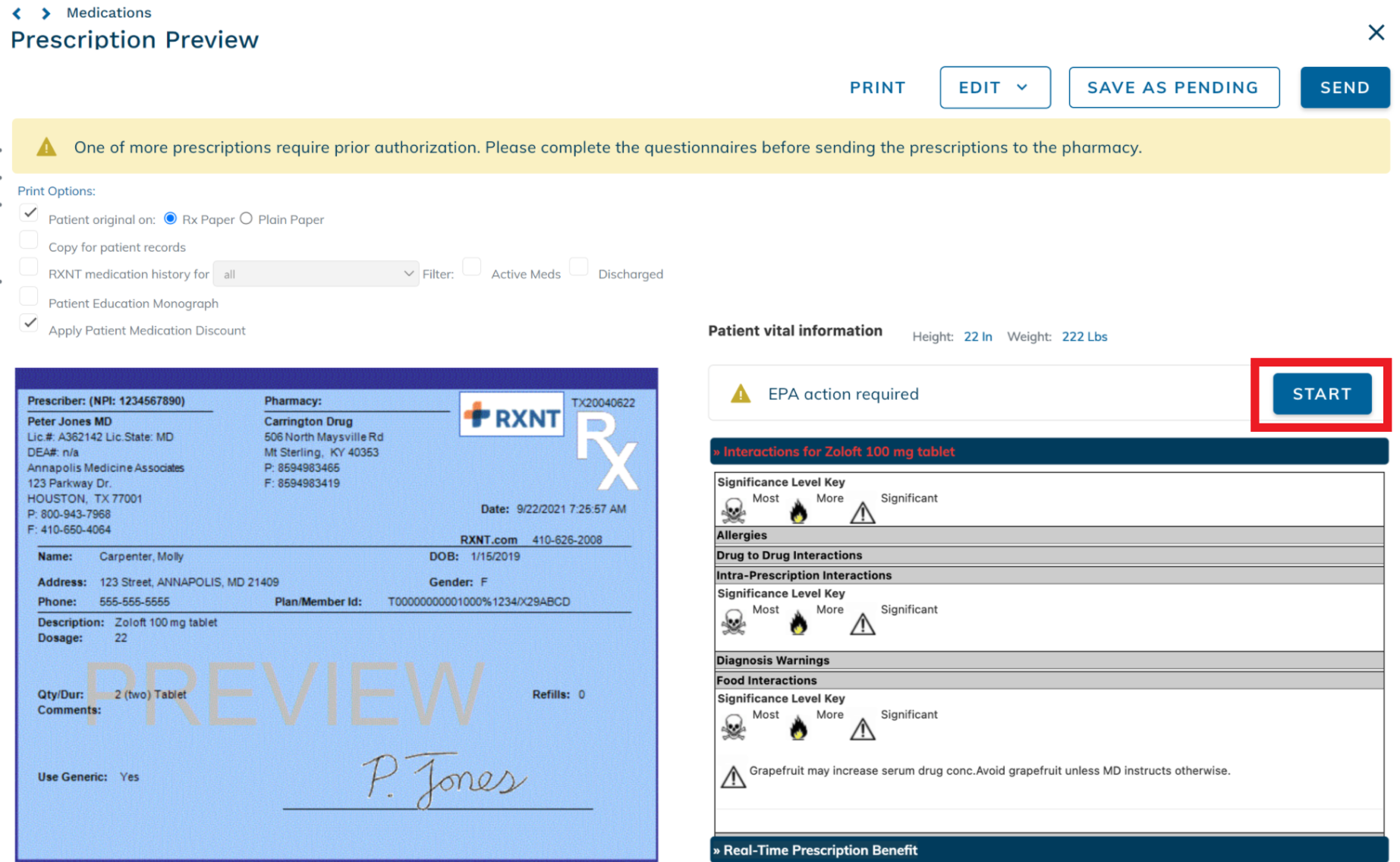The image displays a user interface for a medication prescription preview. At the top, there is a heading labeled "Medication Prescription Preview," accompanied by a set of buttons to the right, including "Print," a drop-down menu labeled "Edit," and another button that states "Save as Pending." Additionally, a prominent blue button labeled "Send" is present.

Beneath these controls is a light brown notification box featuring a yellow triangle icon. The text within the box reads, "One or more prescriptions require prior authorization. Please complete the questionnaire before sending the prescription to the pharmacy."

Further below, there are some smaller, less legible text entries, a few of which are marked with checkmarks.

At the bottom of the image, there is a light blue box outlined with a dark blue border at the top. This box contains a white rectangle with "RXNT" written in blue letters, accompanied by a gold and blue cross. Inside the white rectangle, the letters "Rx" are positioned on the top right side, while the word "Preview" is written at the bottom in capital pink letters. Finally, the signature "P. Jones" appears on a designated signature line.